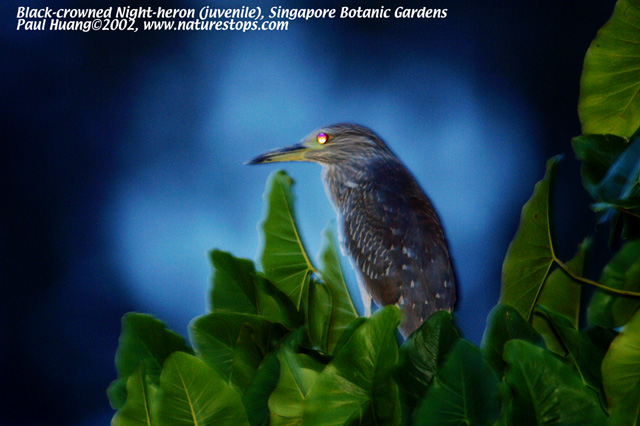This detailed nighttime photograph captures a juvenile Black-crowned Night Heron, as identified by the text in white lettering in the top left corner of the image: "Black-crowned night heron, juvenile, Singapore Botanic Gardens, Paul Huang, Copyright 2002, www.naturestops.com." The bird, primarily gray and black with blue and brown feathers accented by patches of white, is perched among dense green leaves toward the bottom right of the image. Its striking eyes shine with vivid red, orange, and yellow hues. The heron's slender, elongated beak is marked with blue and yellow tones. The background of the photograph features a dark nighttime setting with a soft, misty blue glow surrounded by deep black, suggesting indirect lighting or camera flash. The intricate details of the bird and the atmospheric nighttime composition provide a rich visual experience.